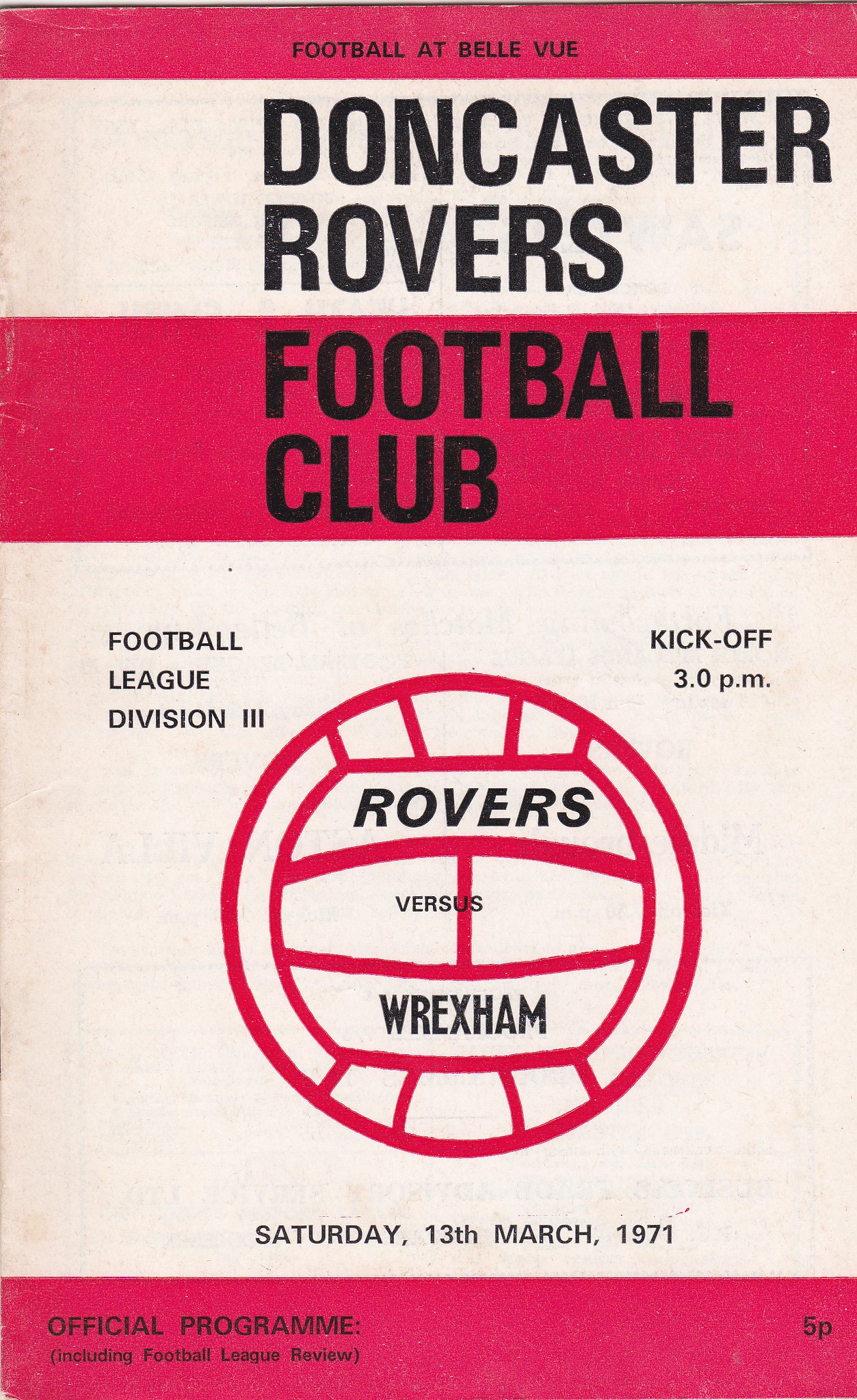The image features a vintage rectangular sports program poster with a background composed of alternating white and pink horizontal stripes. At the top, a thin pink stripe contains the black text, "Football at Belle Vue." Below that, a larger white stripe showcases the bold, black, capital letters "Doncaster Rovers." Following this, a thicker pink stripe displays the black text "Football Club." Centrally positioned on the poster is a pink illustration of a soccer ball, within which it reads "Rovers versus Wrexham" in black. To the top left of the soccer ball, it says "Football League Division 3" in black text, while the upper right side reads "Kickoff 3 p.m." Below the soccer ball, the date "Saturday, 13th March 1971" is inscribed in black. The bottom of the poster features a thin pink stripe; the left side reads "Official Program (including Football League Review)" in black, and the right side denotes the price "5p."